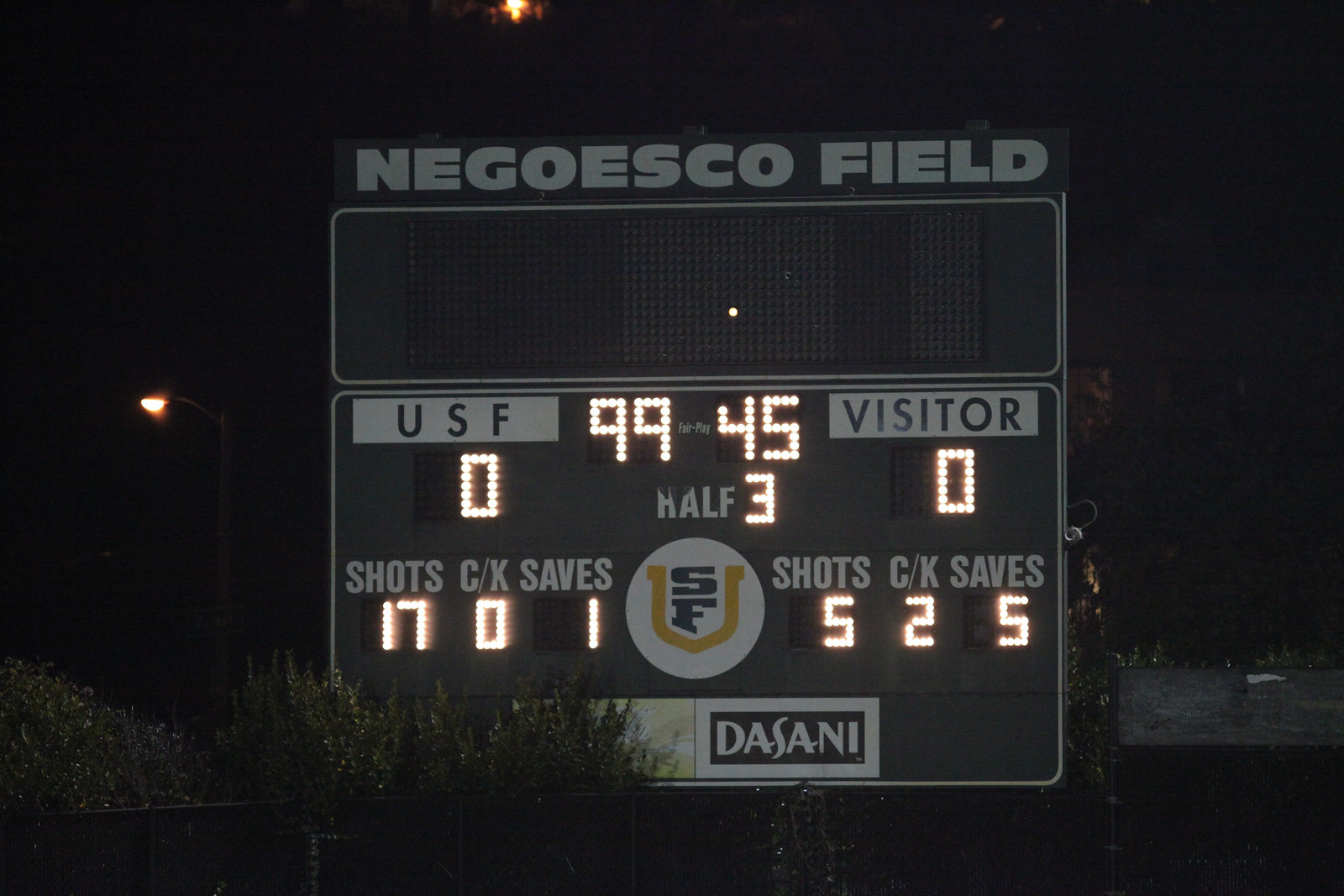The image features an illuminated scoreboard set against a pitch-black night sky at Negoesco Field. The scoreboard prominently displays the scores: USF leading with 99 points against the Visitors' 45. The board indicates it's halftime, showing various in-game statistics, with the teams’ shots, saves, and corner kicks detailed—USF has 17 shots, 0 corner kicks, and 1 save, whereas the Visitors have 5 shots, 2 corner kicks, and 5 saves. The brightly lit display also includes a Dasani Water sponsorship at the bottom. Surrounding the scoreboard, there are visible plants and trees partially covering it from the bottom.